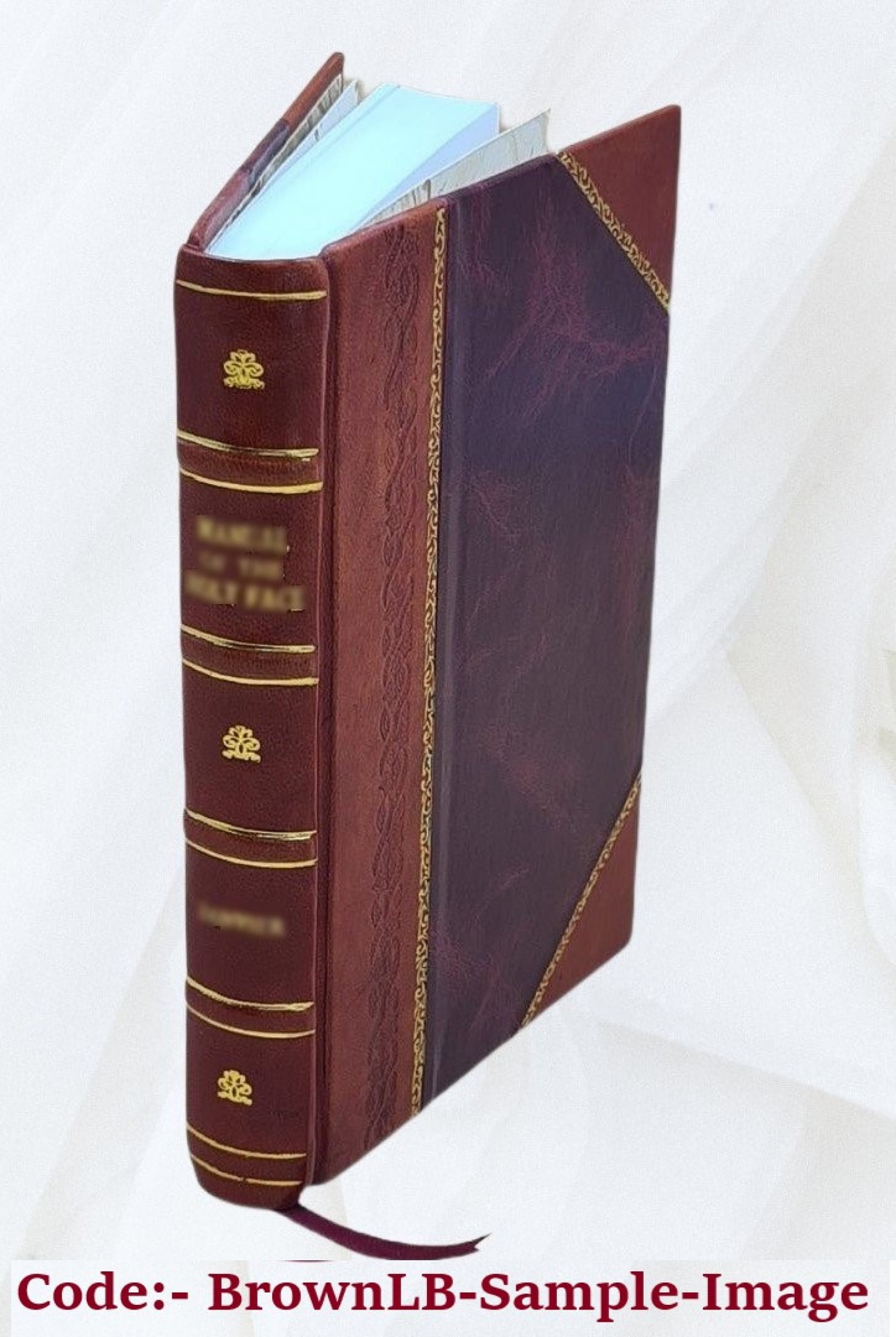This is a photograph of a book with a brown leather cover and spine, displayed upright as if placed on a bookshelf with the spine facing the viewer. The spine is adorned with intricate gold designs, including small trees at the top, bottom, and center, and features the book's title in gold print near the top. The book's pages have a bluish tint and a ribbon bookmark dangles from the bottom. The cover showcases a contrasting purplish leather triangle in the middle, bordered by a black marble-like pattern and maroon leather, all separated by gold trim. The background of the image is a light gray with faint beige shapes that blend into the white backdrop. At the bottom of the image, there is text in dark brown serif font that reads "code: brownLB-sample-image."